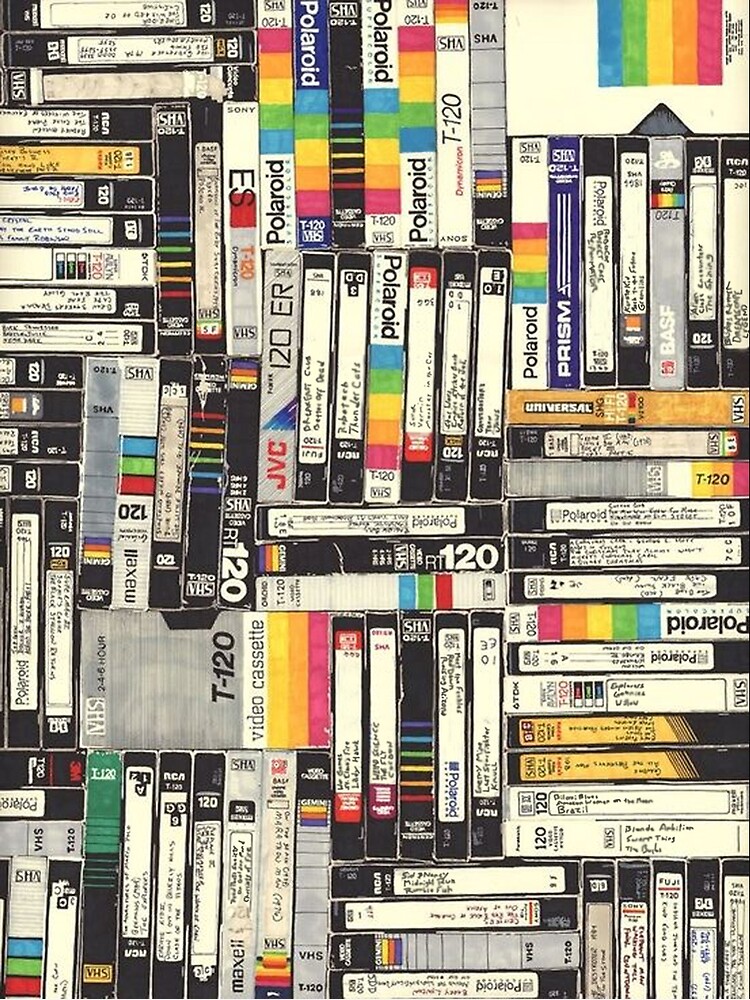The color photograph depicts a diverse and extensive collection of approximately 50 videocassette tapes (VHS), primarily Polaroid brand, distinguished by their characteristic rainbow color strip. The tapes are arranged haphazardly, with some stacked horizontally and others vertically, creating a visually chaotic scene. Nearly all the tapes feature hand-written labels, with titles such as "Blonde Ambition," "Summer Girl," and "Rumor Fest," though many labels are difficult to read due to orientation and handwriting. Common labels include "T-120," suggesting 120-minute tapes, and brands such as JVC, EST, and Prism are also visible. The tapes occupy nearly the entire frame, as if one is looking down upon a shelf filled to capacity with home video recordings.